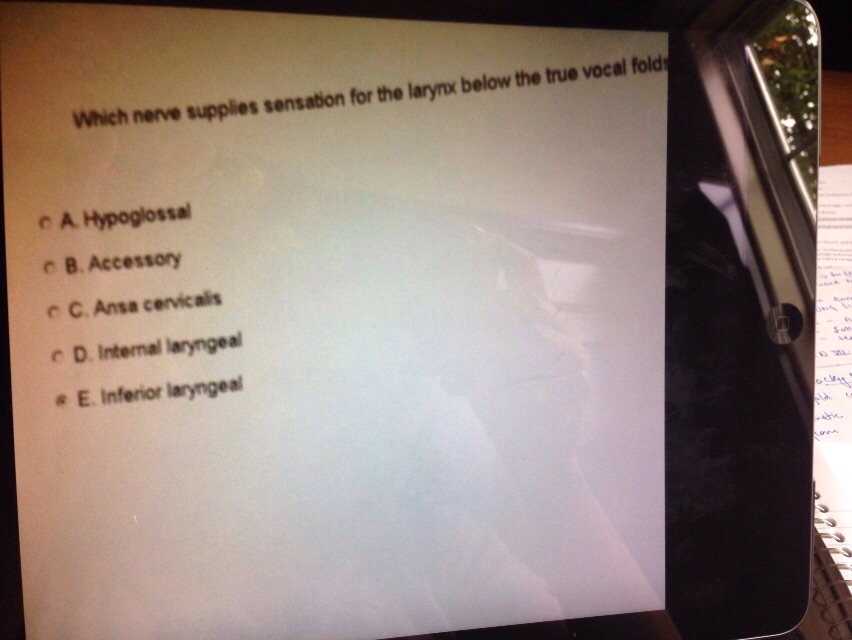The photograph captures an iPad screen laying on its side, with the home button visible on the right. The screen displays a question in black text on a white background: "Which nerve supplies sensation for the larynx below the true vocal folds?" with multiple-choice options: A) Hypoglossal, B) Accessory, C) Ansa Cervicalis, D) Internal Laryngeal, and E) Inferior Laryngeal, with the option E selected, indicated by a dot next to it. Visible in the iPad's reflection are a window and the photo taker. To the right of the iPad, a spiral notebook with handwritten notes sits on what appears to be a wooden table. The notebook paper is white.